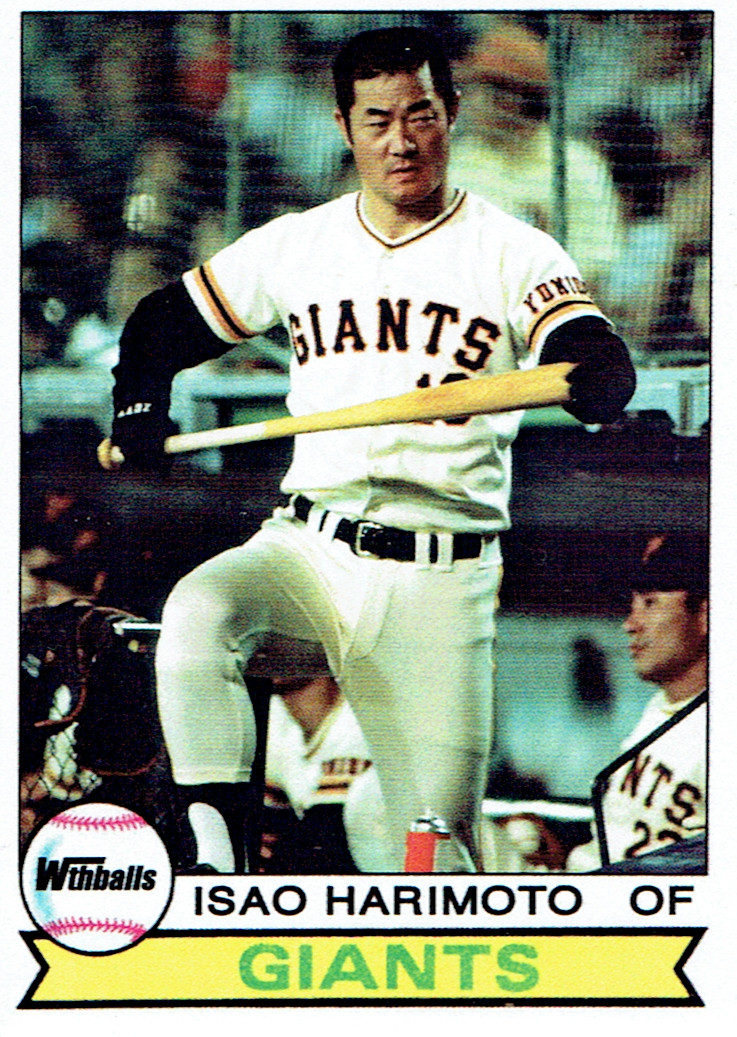This detailed image illustrates a baseball card featuring Isao Harimoto, an outfielder for the San Francisco Giants, identifiable by the "Giants" text boldly adorned in green on a yellow ribbon. Harimoto, possibly of Asian descent, is captured in an older photograph: He sports a classic uniform with the iconic "Giants" team name emblazoned in orange and black on his white jersey, which also features distinct orange and black stripes on the shoulders. Underneath his jersey, he wears black long sleeves and pairs the ensemble with white pants cinched by a black belt. Harimoto is poised holding a brown wooden bat, seemingly walking out of the dugout, further adding to the sense of authenticity and action in the scene. The background teems with fans in the stands, and another player can be seen situated in the dugout's lower right corner. Complementing the nostalgic feel of the card, the phrase "WTHBALLS" is playfully integrated into the design along with a baseball logo, cementing the image as a piece of memorabilia or an advertisement celebrating Harimoto's role in the Giants' storied history.